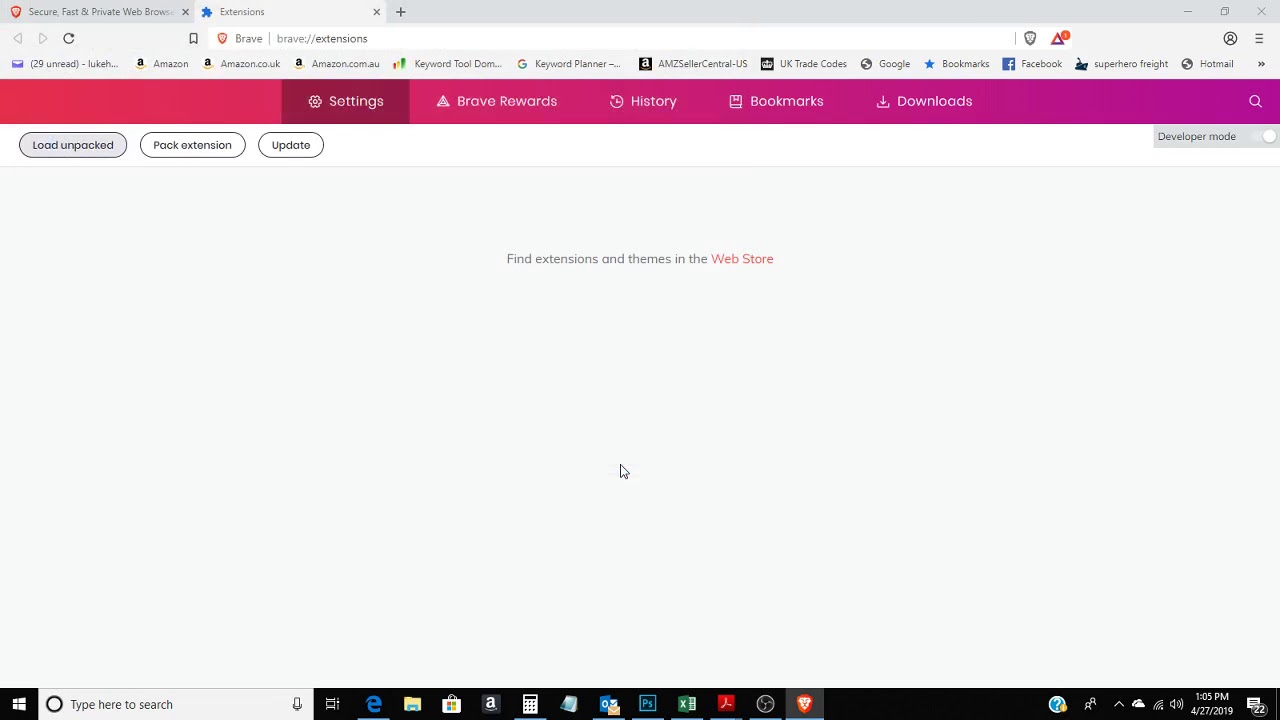This image is a detailed screenshot from a computer's desktop. At the top of the screen, several website browser tabs are open. The first tab is labeled "Secure Fast and Private Web Browser" and features a red logo. The second tab is labeled "Extensions" and displays a blue puzzle piece icon next to it. The tabs belong to the Brave browser, as indicated by the red and purple navigation bar underneath, which includes: Settings, Brave Rewards, History, Bookmarks, Downloads, and a white magnifying glass for search options. "Developer mode" features prominently, providing options such as "Load Unpacked", "Hack Extension", and "Update."

Below the navigation bar, the main content of the page displays "Find Extensions and Themes in the Web Store."

At the bottom of the screen, the taskbar is visible, featuring several icons. On the left side, there’s the Windows icon with a "Type to Search" box next to it, followed by quick access icons for various programs: Microsoft Edge, a Files folder, the Microsoft Store, Amazon, Calculator with a white icon, Notepad, Microsoft Outlook, Adobe Photoshop (PS), Microsoft Excel (green icon), Adobe (likely Acrobat), and an icon resembling a small black circular fan. There is also an orange lion icon, which represents the Brave Browser.

The taskbar also includes system indicators for Wi-Fi and volume control. The time is displayed as 1:05 PM, and the date is noted as April 27, 2019. Additionally, there is a notification icon with the number 22 indicating unseen notifications.